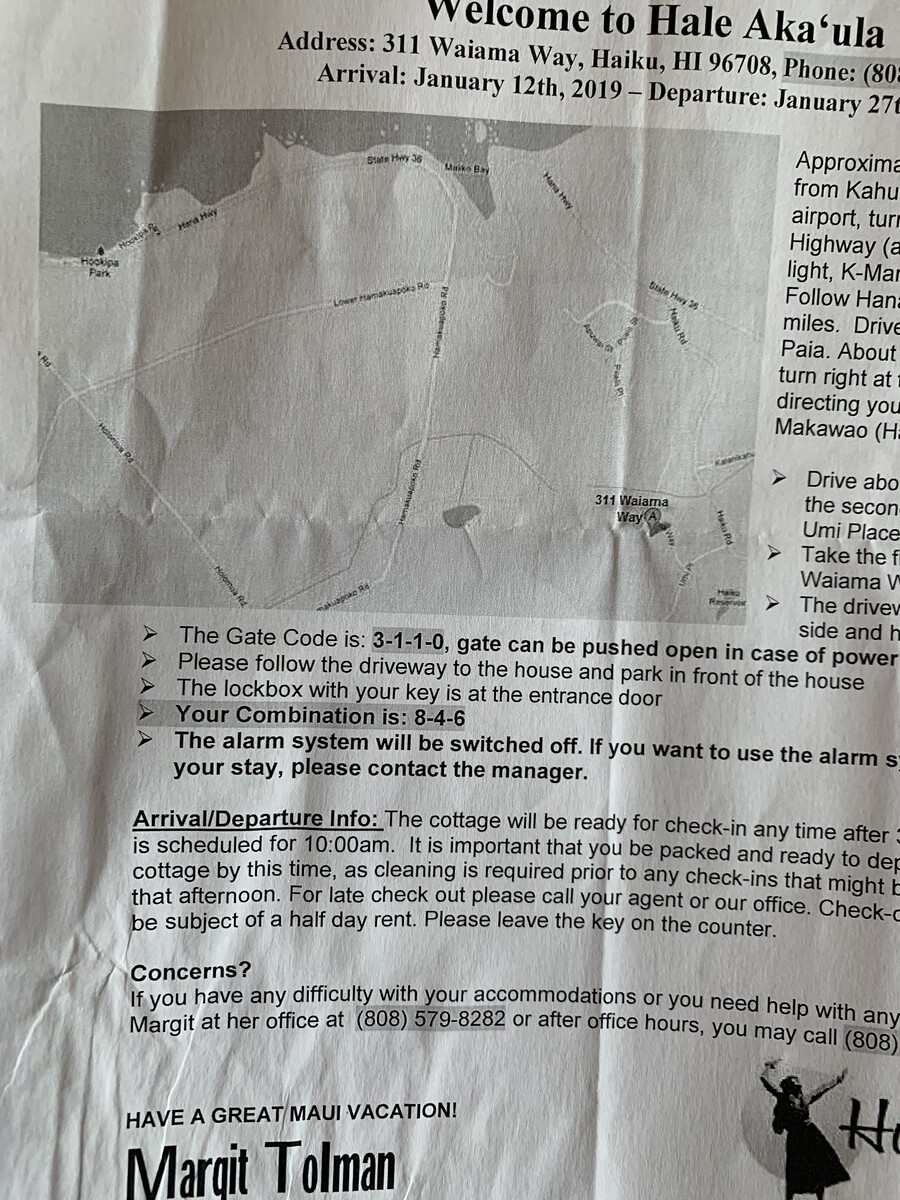The image is a close-up of a crinkled paper that appears to be a welcome notice for Hale Aka'ula, likely a cottage or bed and breakfast in Haiuka, Hawaii. At the top, in prominent black lettering, the text reads: "Welcome to Hale Aka'ula, Address: 311 Wai'ama'a Way, Haiuka, Hawaii." Although the full phone number is partially cut off, a visible number at the bottom reads (808) 579-8282. Below this heading is a black-and-white map illustrating the local streets and outlining where the water meets the land, though the text on the map is too small to read clearly. Following the map are several important bullet points: the gate code is 3110, and it mentions that the gate can be pushed open in case of a power outage. Guests are instructed to follow the driveway to the house and park in front. The lockbox at the entrance has a key combination of 846, with the alarm system being switched off unless you contact the manager. There is also specific information about arrival on January 12, 2019, and departure on January 27, with further instructions to reach out to the manager during their stay for any concerns. The bottom of the notice, framed by a once-folded crease, asks visitors to "Have a great vacation" and features a signature from Markit Thalman, along with a small black-and-white image of a person.